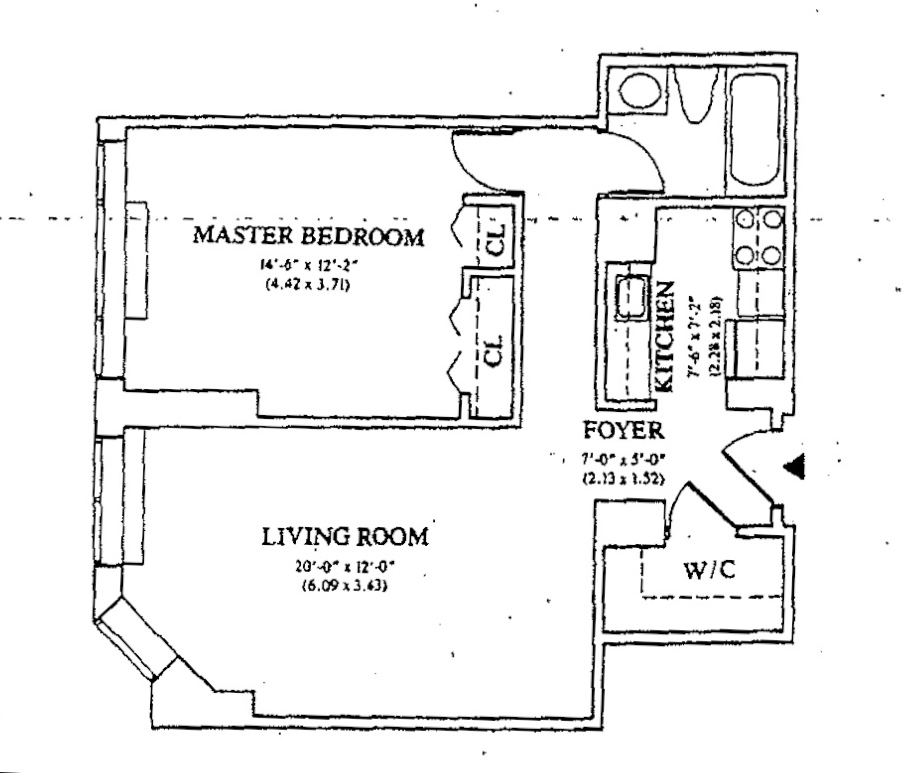The image displays a detailed floor plan of a building's first floor. Prominently featured is a spacious master bedroom measuring 14.6 by 12.2 feet, which includes a window and two closets for ample storage. Adjacent to the master bedroom is a bathroom. The expansive living room, occupying 20 by 12 feet, serves as a central gathering space and leads directly to the kitchen via a 7 by 5 feet foyer. The foyer itself is well-organized with a closet on the right side and the kitchen on the left. The overall layout forms a basic block shape, efficiently arranging the master bedroom, living room, and kitchen for optimal functionality.